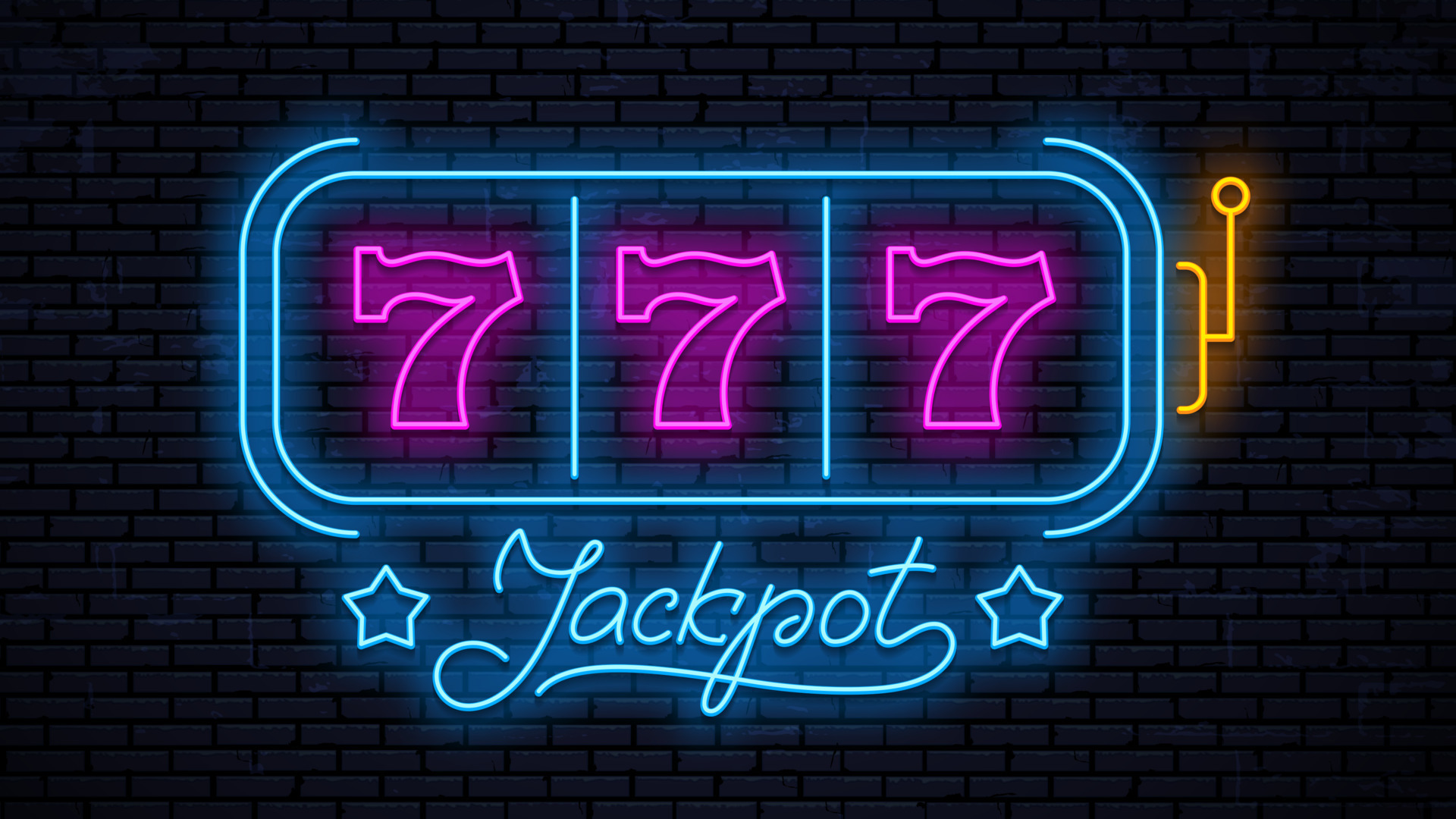This is an image of a neon sign designed to resemble a classic slot machine, digitally created and displayed on a black brick wall. The vibrant sign features the number "777" in hot pink or bright purple, encased within a horizontally rectangular frame with rounded corners. Surrounding this frame is an additional layer of rounded rectangles in blue. Each "7" is separated by a blue line. Below the sevens, the word "Jackpot" is written in cursive, also in blue, flanked by two blue stars on either side. On the right side of the sign, there's a neon yellow lever, reminiscent of the pull handle on traditional slot machines, further enhancing the casino theme. The overall composition vividly contrasts against the dark, almost purple-hued brick background, emphasizing the bright, multi-colored neon elements.